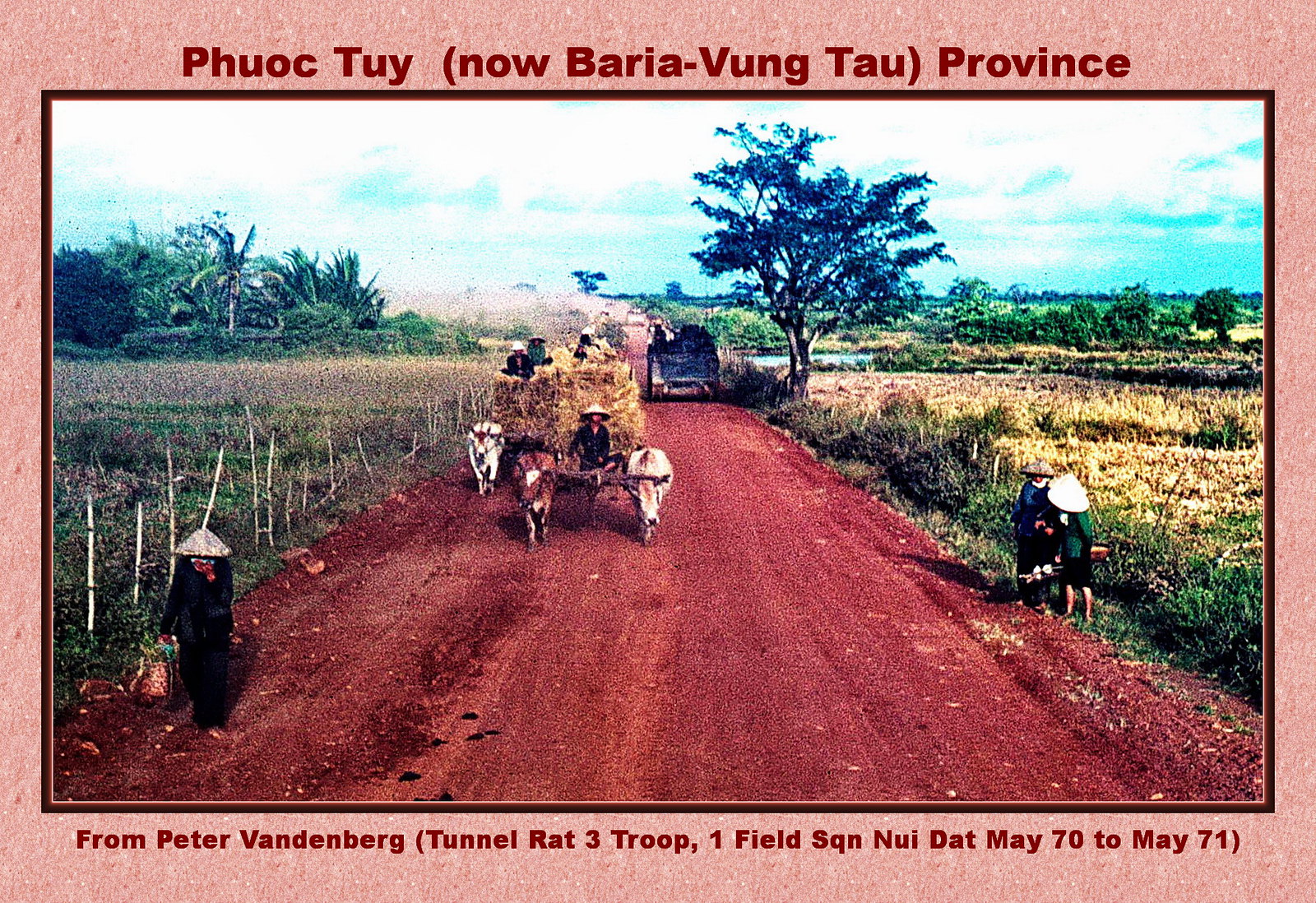This photograph captures a vibrant scene on a wide dirt road in rural Vietnam, flanked by green fields and sporadically dotted with trees. Central to the image is a cart being pulled by three cattle, laden with numerous bales of hay. The cart driver, wearing a traditional conical hat, is accompanied by a couple of passengers perched atop the hay. Various workers are visible along the road; on the left, a solitary figure walks, while on the right, two individuals chat animatedly. Almost everyone in the scene dons conical hats, adding to the cultural authenticity of the depiction. Surrounding the image is text indicating the location and date: "Phuoc Tuy, Nauberia, Vung Tau, Providence, from Peter Vanderburgh, Tunnel Rat 3 Troop, Onefield, SQN, Nui, Dat, May 72, May 71."